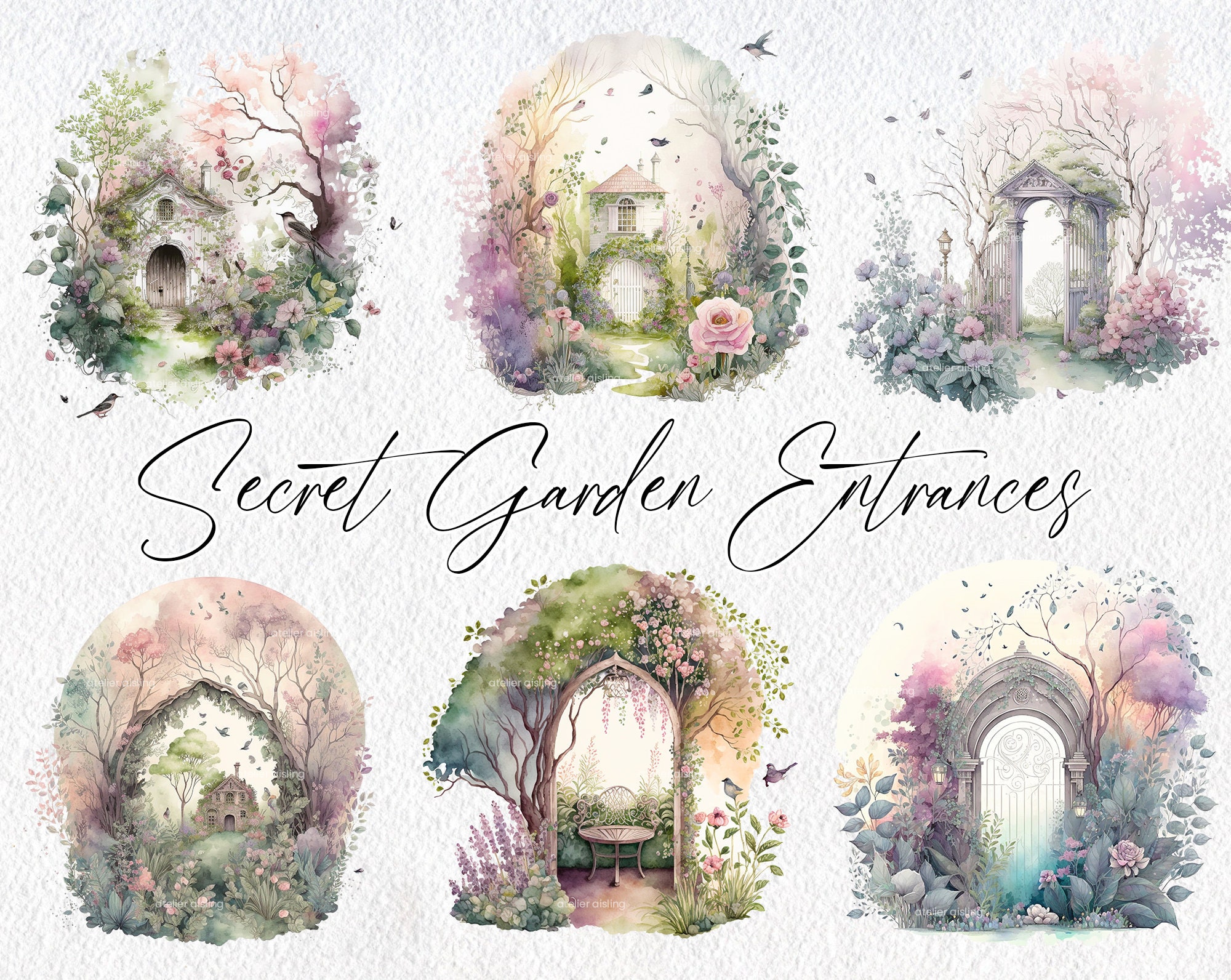This image features six different paintings of garden entrances, displayed on a textured, canvas-like background that you can almost feel the indentations on. In the center, in elegant italics, it reads "Secret Garden Entrances." The background is predominantly blue with a subtle pattern running through it, enhancing the artistic ambiance. The paintings are arranged in two rows, three per row, each illustrating unique artist renditions of secret garden gateways.

From left to right, top to bottom, the top left painting shows a charming little house with pastel pink, purple, and green hues adorning the scene. The second image in the top row features another quaint house amidst a garden, while the top right showcases an archway gazebo surrounded by colorful flowers. On the bottom row, the leftmost image depicts another house amidst vivid pink and purple blooms. The middle one presents an archway with a table in the center, enveloped by lush greenery and delicate flowers. The bottom right features yet another arch, possibly made of glass, framed by intricate floral designs. The entire collection is rich in pastel colors, prominently featuring soft pinks, purples, and greens, with occasional appearances of birds adding a lively touch to the serene settings.